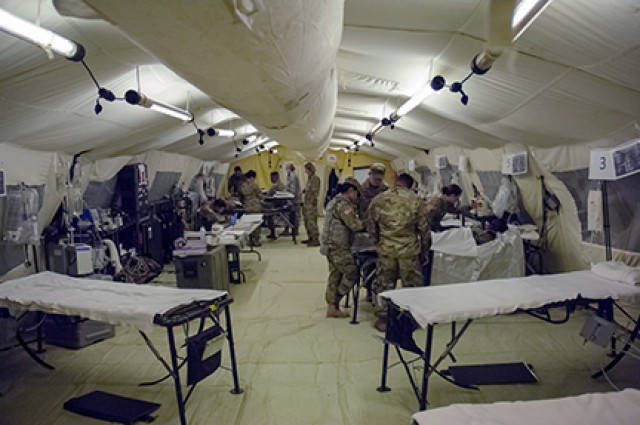The image depicts a color photograph of a temporary military field hospital, captured in landscape orientation. The scene is centered on a central walking path flanked by rows of narrow hospital beds with white sheets and folding metal legs. The facility appears to be housed inside an inflatable, tent-like structure, indicated by the white, arced fabric ceiling and walls. A prominent large pipe runs along the middle of the ceiling, flanked by rows of overhead fluorescent lights. On the ground are several foldable chairs covered with white cloths, and at the foot of each bed are bags presumably for storing notebooks or other items. The right center of the image is occupied by several individuals in camouflage uniforms attending to a patient at one of the tables. In the far end of the image, another team of soldiers can be seen working around a table, surrounded by various pieces of medical equipment. The photograph is a detailed representation of a bustling, makeshift medical facility in a military context.